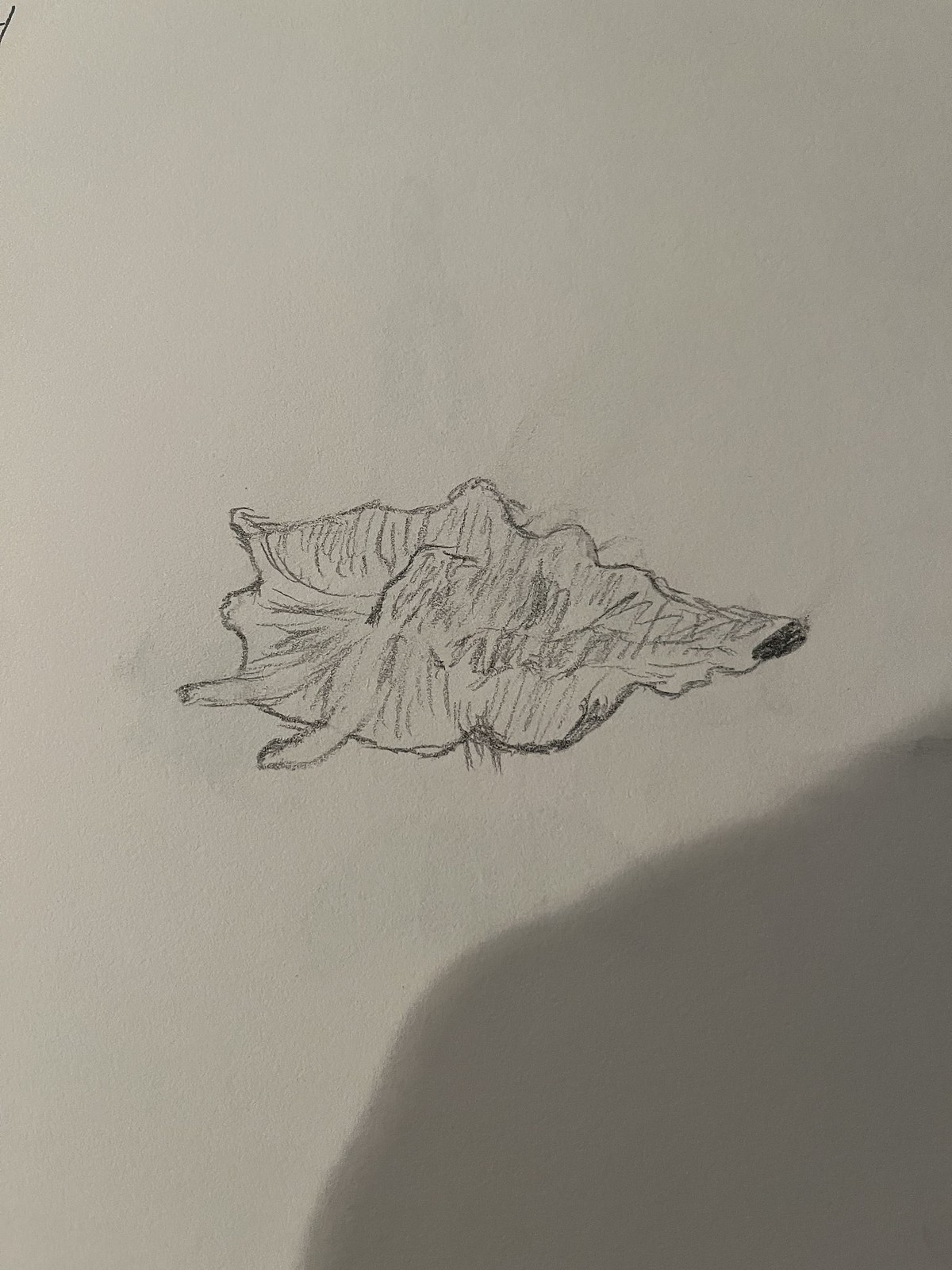The image depicts a pencil line drawing on what appears to be a white piece of paper, although the lighting gives the paper a slightly tan hue. The drawing, which is basic and somewhat ambiguous, resembles a seashell viewed from the top. It features various lines indicating texture, with the left side appearing fatter and the right side skinnier. There are smudges on the left and lower parts of the paper, suggesting erasures and redrawing. The background includes the shadow of the person who took the photo, noticeable in the lower right-hand corner, indicating the presence of a light source behind them. Overall, the drawing is a simple, hand-drawn sketch with subtle imperfections and shading variations.